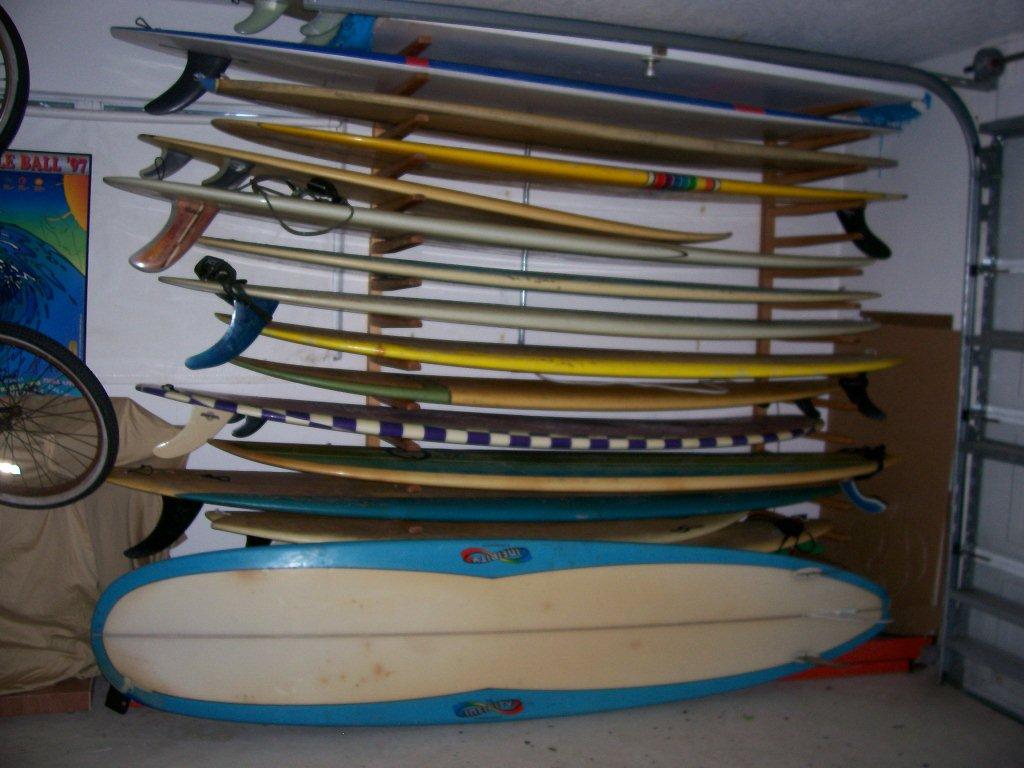This image captures a detailed scene inside a car garage. Dominating the view is a rack of surfboards, positioned directly to the left of the garage door, which features visible tracks and railing. The surfboards are varied in size and color, including white, light blue, dark blue, purple, orange, yellow, gold, and red, all stored horizontally. On the floor in front of the rack lies a white surfboard with a blue edge and fins facing towards the viewer, adorned with an Infinity logo on both sides. To the left of the frame, a bicycle can be seen hanging from the ceiling, with just the wheels and spokes visible. Behind the bike, a poster hangs on the wall, displaying an image predominantly blue, depicting the top of the Earth with the sun in the top right corner. The poster bears the text "Ball 97" in red, though some text is cut off. The wall of the garage is white, and the floor features a gray and white dotted texture. There is also mention of a painting and a tarp beneath it on the wall to the left.